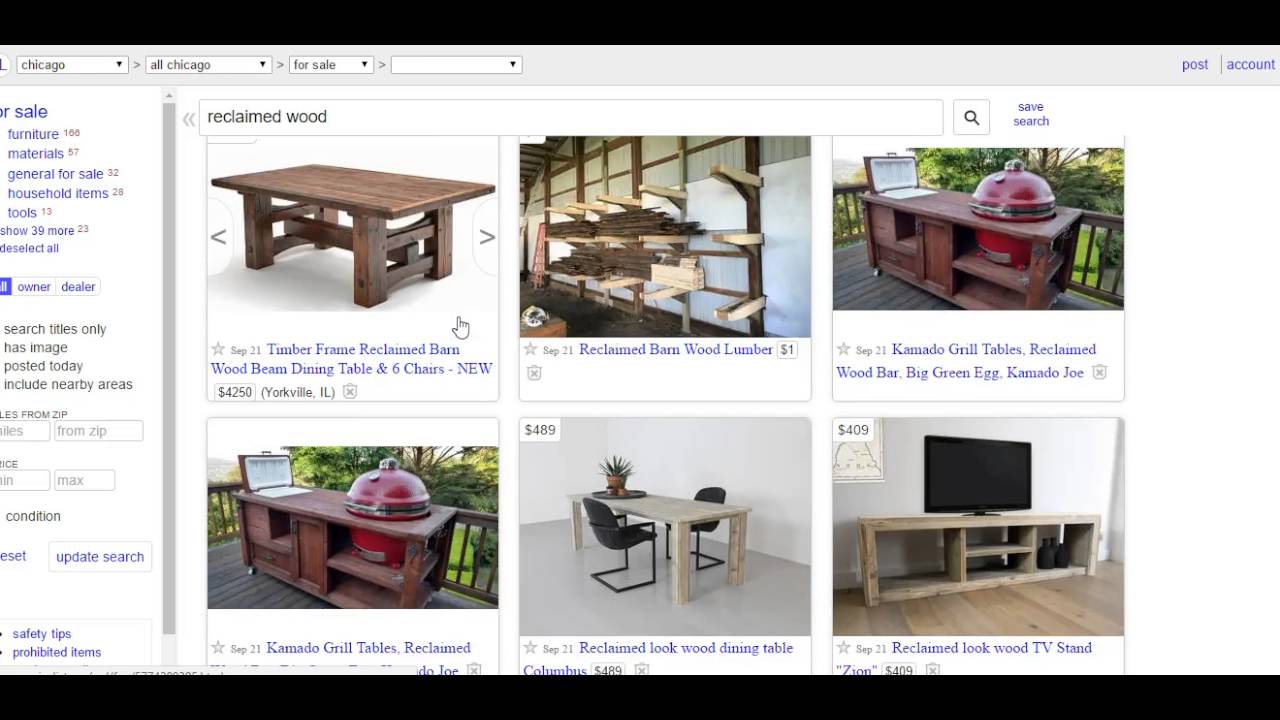Screenshot of an online marketplace page titled "Reclaimed Wood". The page features six individual images, each showcasing distinct products made from reclaimed wood. 

1. The top left image displays a substantial picnic table with a plain wood plank surface on sturdy wood legs. The caption reads "Timber Frame, Reclaimed Barn Wood, Beam Dining Table, and Six Chairs, New, $4,250, Yorkville, Illinois." Notably, the image does not include the advertised chairs.

2. The top center image features stacks of wood neatly displayed, captioned "Reclaimed Barn Wood Lumber."

3. The top right image showcases a rustic grill table, identified as "Kamado Grill Tables, Reclaimed Wood Bar, Big Green Egg, Kamado Joe." The table sits on a wood-planked patio and is surrounded by a wooden fence and lush greenery.

4. The bottom left image mirrors the top right image, showing the same Kamado Grill Table set on a wood-planked patio, with a wooden fence and verdant shrubbery in the background.